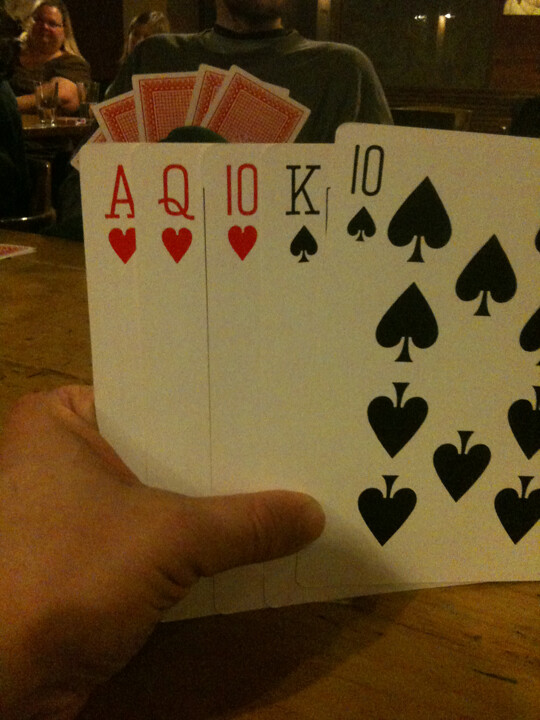In this evocative photograph captured in portrait mode, the perspective is from someone engaged in a game of poker. The central focus is on the player's hand, confidently displaying five cards: the Ace of Hearts, the Queen of Hearts, the Ten of Hearts, the King of Spades, and the Ten of Spades, all poised over a rustic wooden table. Directly across, a man in a casual t-shirt clutches his own hand of cards, their red backs hinting at the hidden strategies within. Further in the background, a heavyset woman with long blonde hair and glasses sits nursing a drink; her short-sleeved shirt adds to her relaxed demeanor. She is engaged in conversation with another young woman seated beside her. The ambient lighting is dim, casting a cozy yet mysterious atmosphere, suggesting the setting is a bar or a club during twilight hours.